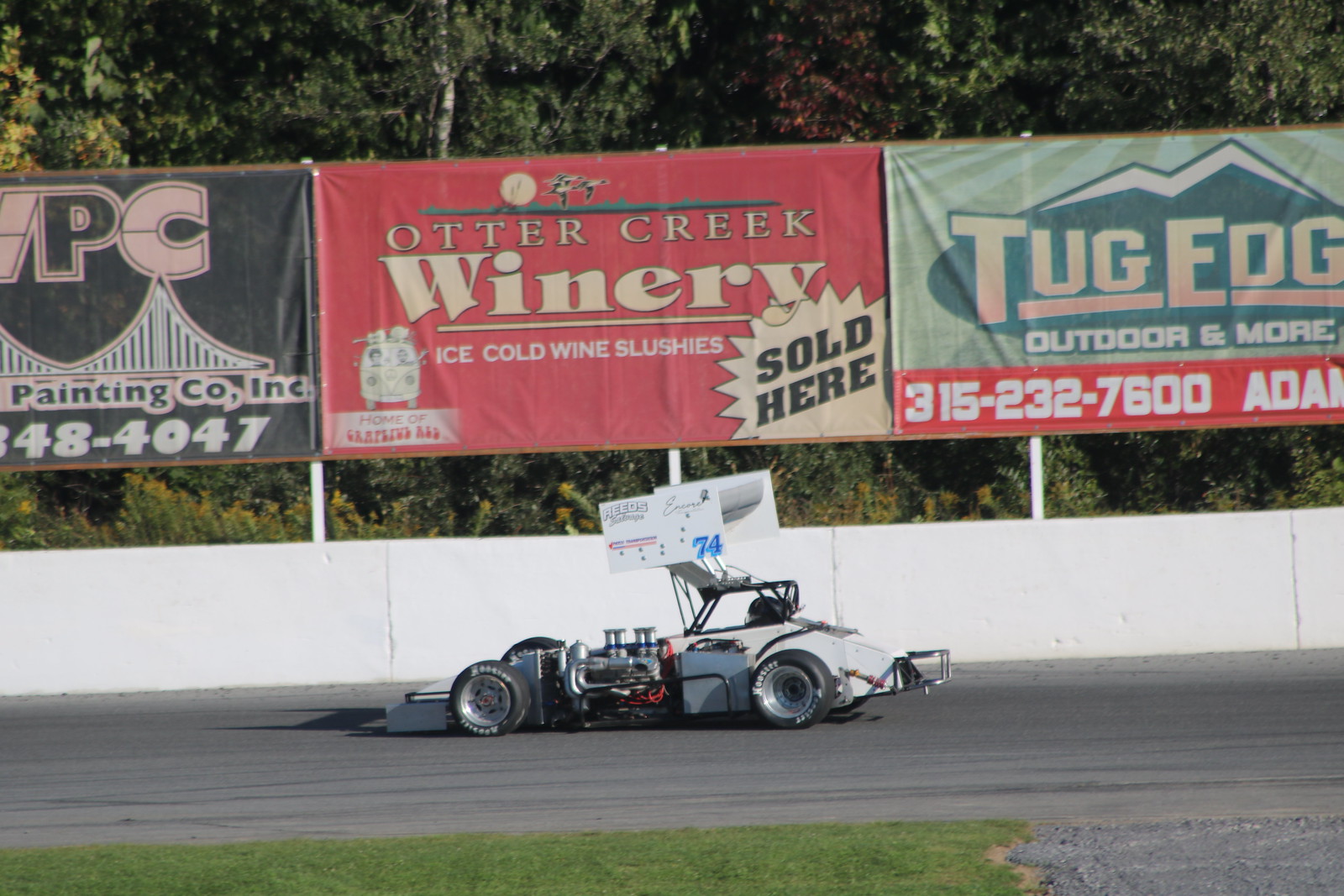The image depicts a sleek, open-seating drag race car on a well-maintained, gray racetrack. The car, characterized by its exposed engine and elevated front wheels, is positioned on the pavement with a visible number tag marked "74" hovering above it. Behind the car stands a white barrier wall adorned with various advertisements. To the left, there is a black banner likely promoting a painting company. Dominating the center is a red banner for Otter Creek Winery, advertising "ice cold wine slushies sold here." On the right, a green and white banner for Tug Edge Outdoor and More includes a phone number. Further in the background, lush green trees frame the scene, providing a contrast to the industrial elements of the racetrack.